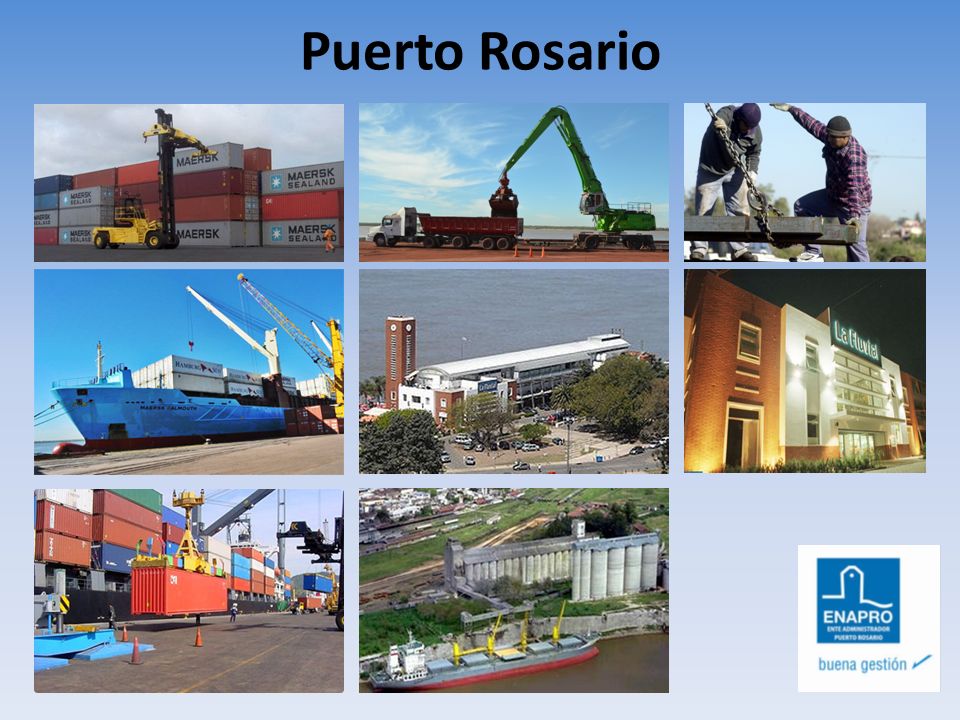The image titled "Puerto Rosario" features a blue-bordered slide showcasing eight detailed photographs, emphasizing the bustling activity and infrastructure of the port. The top left photograph displays Merce shipping containers, while the top center focuses on heavy machinery and trucks. Adjacent to it on the right, there are construction workers accompanied by beams. Positioned below, another image captures a ship equipped with cranes operating near a large building by the sea. This prominent building, labeled "La Fluvial," resembles a hotel and stands out in the middle of the slide. The bottom left photo continues the theme of shipping with more containers, while the bottom center shows another vessel docked near the shore alongside some buildings. Concluding the montage on the bottom right, the slide features the logo for Enapro with the text "Buena Gestión." The amalgamation of these visuals underscores the extensive shipping, construction, and logistical operations pivotal to Puerto Rosario.